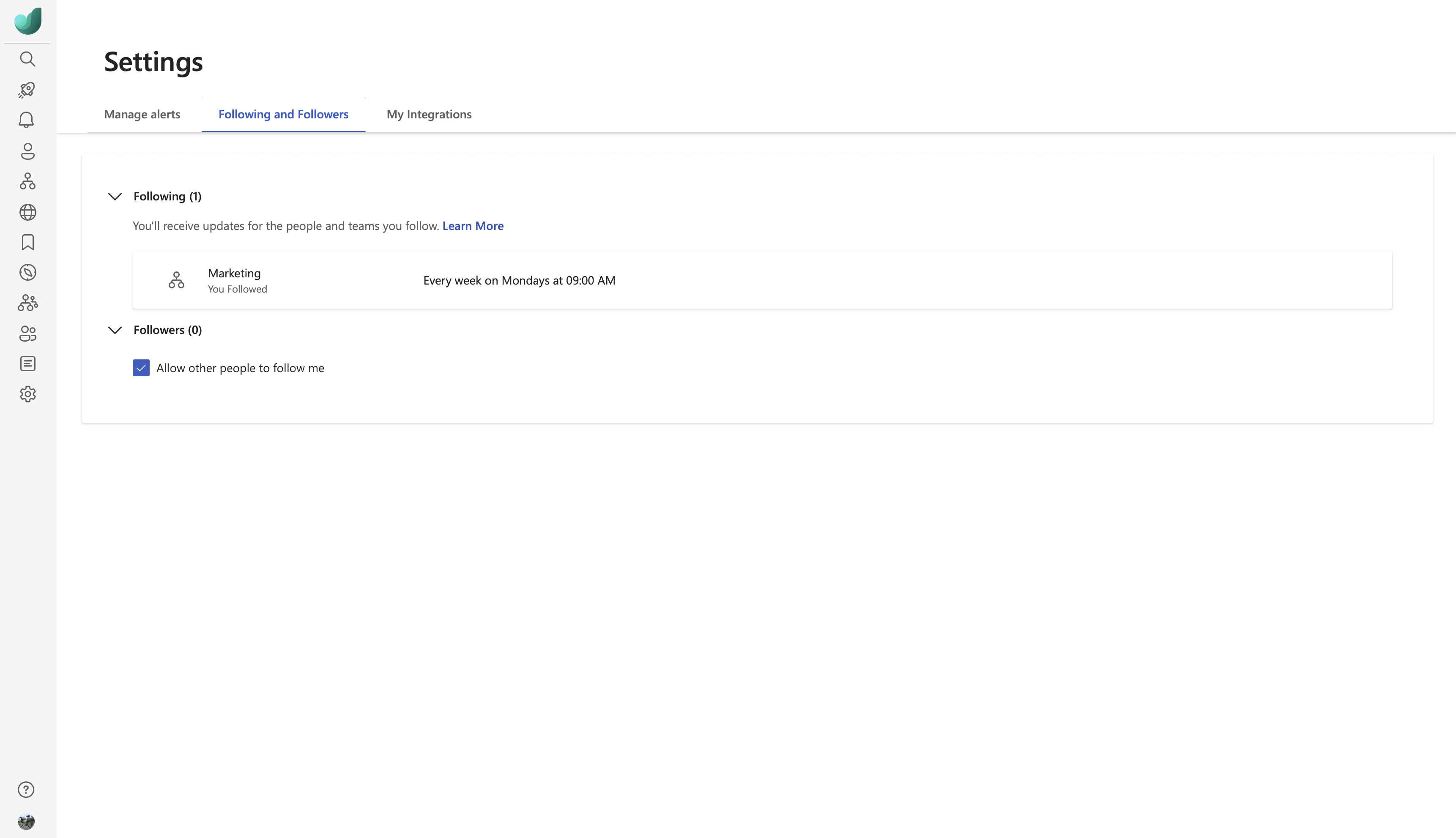**Detailed Caption:**

This image is a landscape-oriented screenshot featuring a predominantly white background. On the left side, there is a vertical gray sidebar extending from the upper left to the lower left corner. At the top of this sidebar, there is an unusual teal-colored icon resembling a bird. Below this icon, the sidebar contains various icons arranged in a vertical sequence: a magnifying glass (search), a rocket, a bell (notifications), a person (profile), a share symbol, a globe, a bookmark, and an icon that resembles a timer. The settings gear icon is positioned near the bottom. In the bottom-left corner of the sidebar, there is a question mark enclosed in a circle, potentially indicating help or information, accompanied by what appears to be an avatar.

In the main section to the right of the sidebar, the title "Settings" is displayed prominently at the top in dark black text. Below this title, there are several tab headers: "Manage Alerts," "Following and Followers," and "My Integrations." The "Following and Followers" tab is highlighted in blue and underlined, indicating it is currently selected.

Within this tab, there is a section heading "Following" with a downward-pointing arrow and a parenthetical note indicating "(1)." This section explains, "You'll receive updates for the people and teams you follow." Below this, in blue text, there is a "Learn More" link, suggesting additional information is available.

The next section is labeled "Marketing," which has a note stating that updates are followed every Monday at 9 a.m. Below this, it indicates that the user is currently following "Marketing."

The following section is titled "Followers" with a count of "0," and it includes a setting option to "Allow other people to follow me."

Overall, this screenshot pertains to settings for notifications related to followers and following activities.